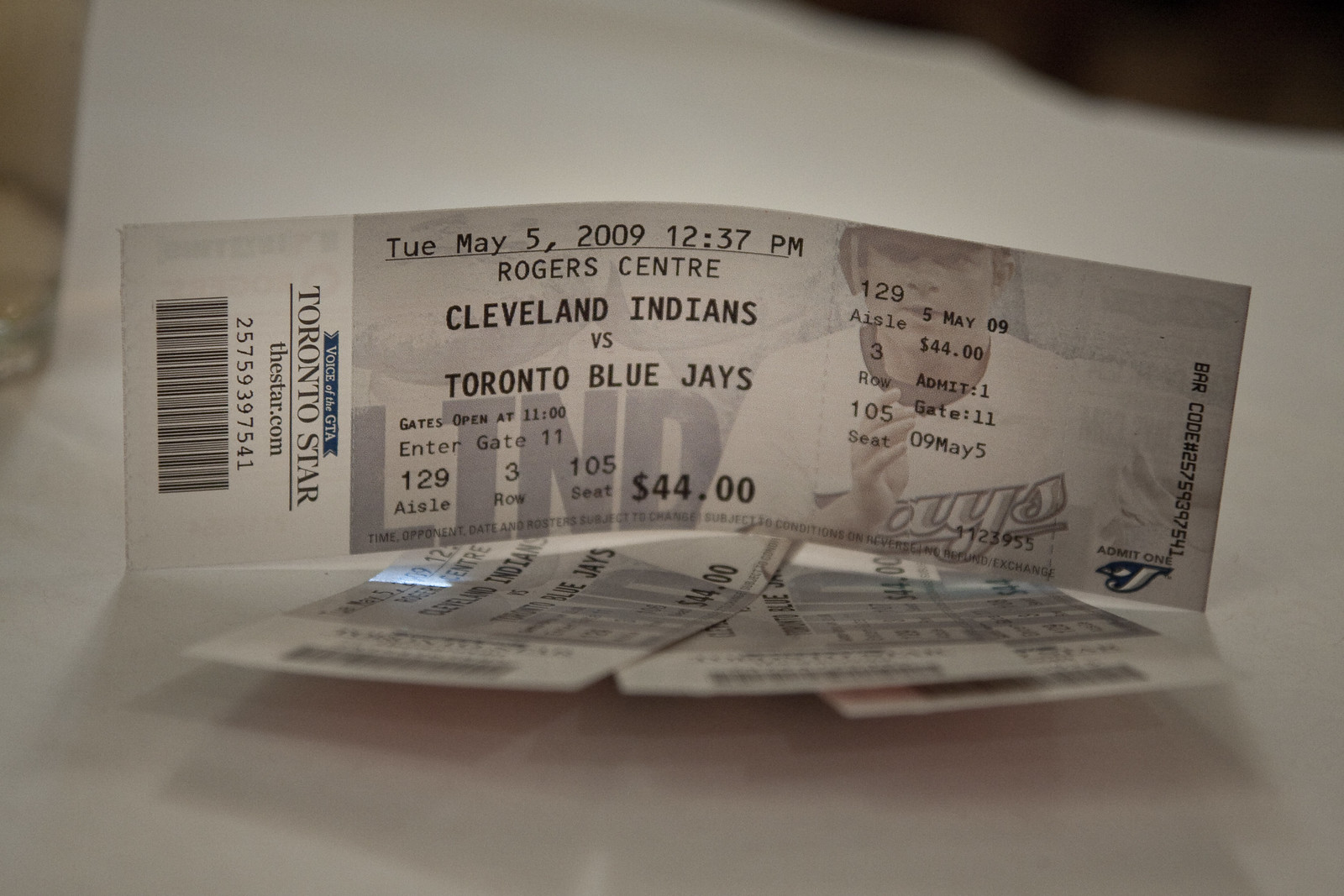This photograph features four baseball game tickets, prominently displaying details for a matchup between the Cleveland Indians and the Toronto Blue Jays at Rogers Center on Tuesday, May 5th, 2009, with the game scheduled to start at 12:37 p.m. Three of the tickets are laid flat, while one is clearly visible and upright. Each ticket, priced at $44, is adorned with the image of a Blue Jays player in the background, subtly incorporated to ensure visibility of the text. Essential details such as the seating arrangement (aisle 129, row 3, seat 105), gate opening time (11 a.m.), and entry gate (Gate 11) are specified on the ticket. The sponsor, Voice of the GTA Toronto Star, is featured along with their website, thestar.com. Additionally, a barcode and scanner number are present for verification. The tickets are lying on a white piece of paper, casting shadows due to the lighting in the room. The photograph is approximately eight inches wide by six inches tall, devoid of any human presence, focusing solely on the tickets.